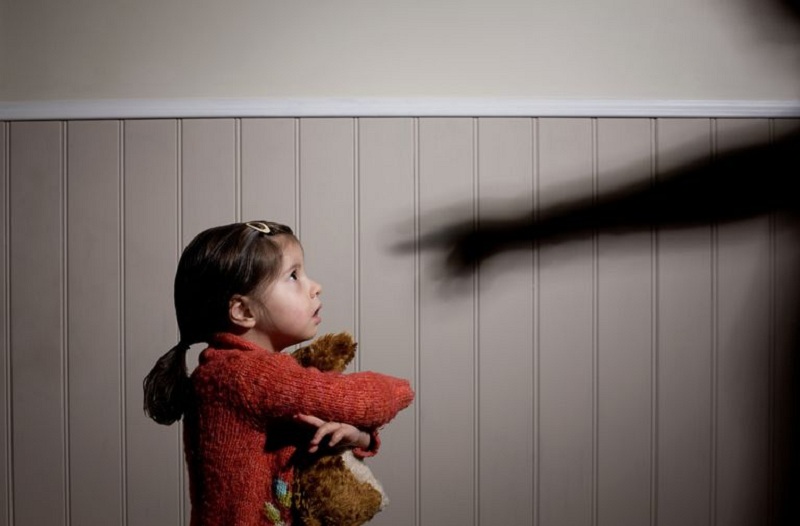In the photograph, a little girl, appearing distraught and scared, clutches a brown teddy bear to her chest. She is positioned on the left side of the image, wearing a red sweater with her brown hair pulled back into a ponytail and a barrette keeping her hair away from her forehead. On the right side of the image, the shadow of an adult, with their index finger pointed accusingly at her, is visible on the wall. The girl’s wide, fearful eyes and slightly open mouth convey her unease as she looks up at the source of the shadow. The background features an eggshell white upper section with a strip of white trim, and below that, a tan-colored wood paneling.